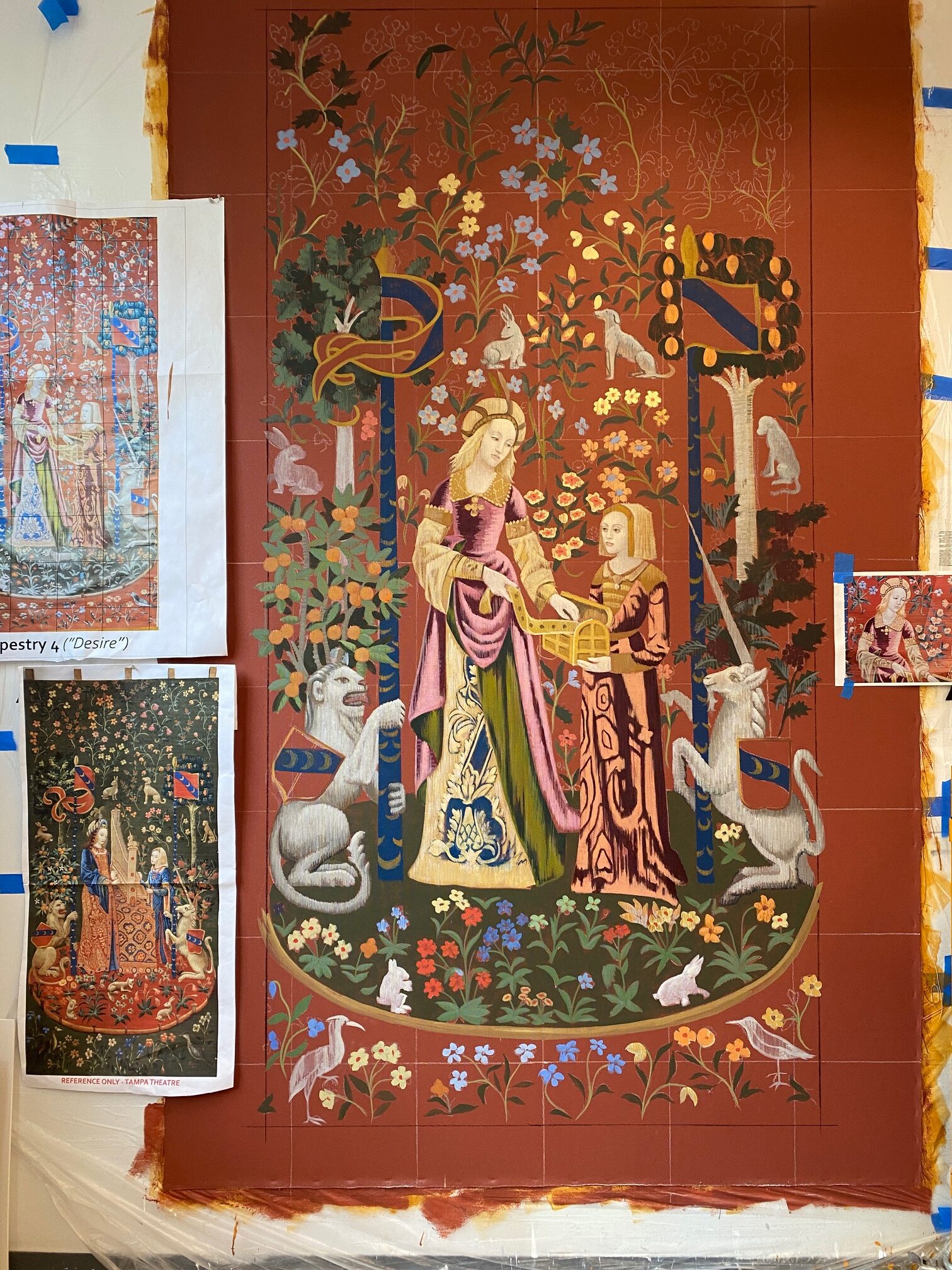This image captures a detailed and ornate painting in progress, mounted on a wall with blue painter’s tape. It portrays a scene reminiscent of the Renaissance or Medieval period, featuring a woman in a pink and white dress with a green accent and a beret-like hat with red outlines. She has yellow hair and is positioned on the left side of the painting, reaching towards a golden treasure chest held by a shorter woman in a red dress with light red tones, who also has yellow hair. The background is filled with an array of colorful, small flowers and rustic tones.

On the left side of the painting, a white lion is depicted with one paw raised, holding up a flag, while on the right side, a unicorn stands upright, also holding a flag. Surrounding these main figures, intricate designs of vines and flowers are evident, creating an ornate border. The painting is overlaid with a protective plastic sheet and features several printed reference images mounted with blue tape, suggesting that this is a carefully arranged work in progress. Additional elements in the scene include birds, bunnies, and smaller statues, enhancing the elaborate garden-like setting of this mural.